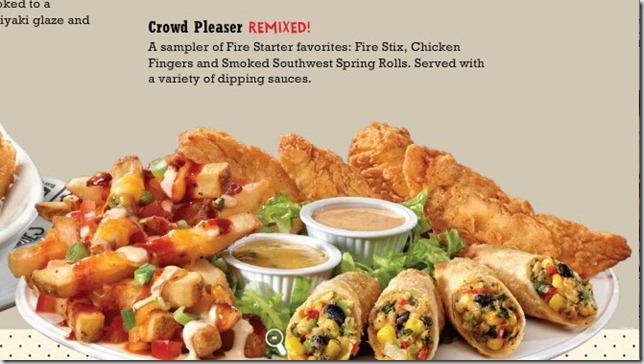The image is a horizontal rectangular advertisement featuring a large white platter brimming with an assortment of delectable foods, set against a beige background. In the center of the platter, two small dishes filled with dipping sauces rest on a bed of lettuce. Surrounding these dishes are three distinct types of appetizer items: crispy egg rolls, sizeable deep-fried pieces that appear to be chicken tenders, and what looks like fully loaded fries. Additionally, on the left side of the platter, there's a scattering of small shish kebab-like vegetables. The bottom of the image features a small polka-dotted banner, while text above it proclaims: "Crowd Pleaser, Remixed - a sampler of Firestarter favorites. Firesticks, chicken fingers, and smoked southwest spring rolls, served with a variety of dipping sauces." The plate is mostly centered but positioned lower in the frame, and the color palette includes tan, black, red, white, brown, yellow, and orange. This appears to be part of a broader ad, possibly the side of a box or a promotional flyer.